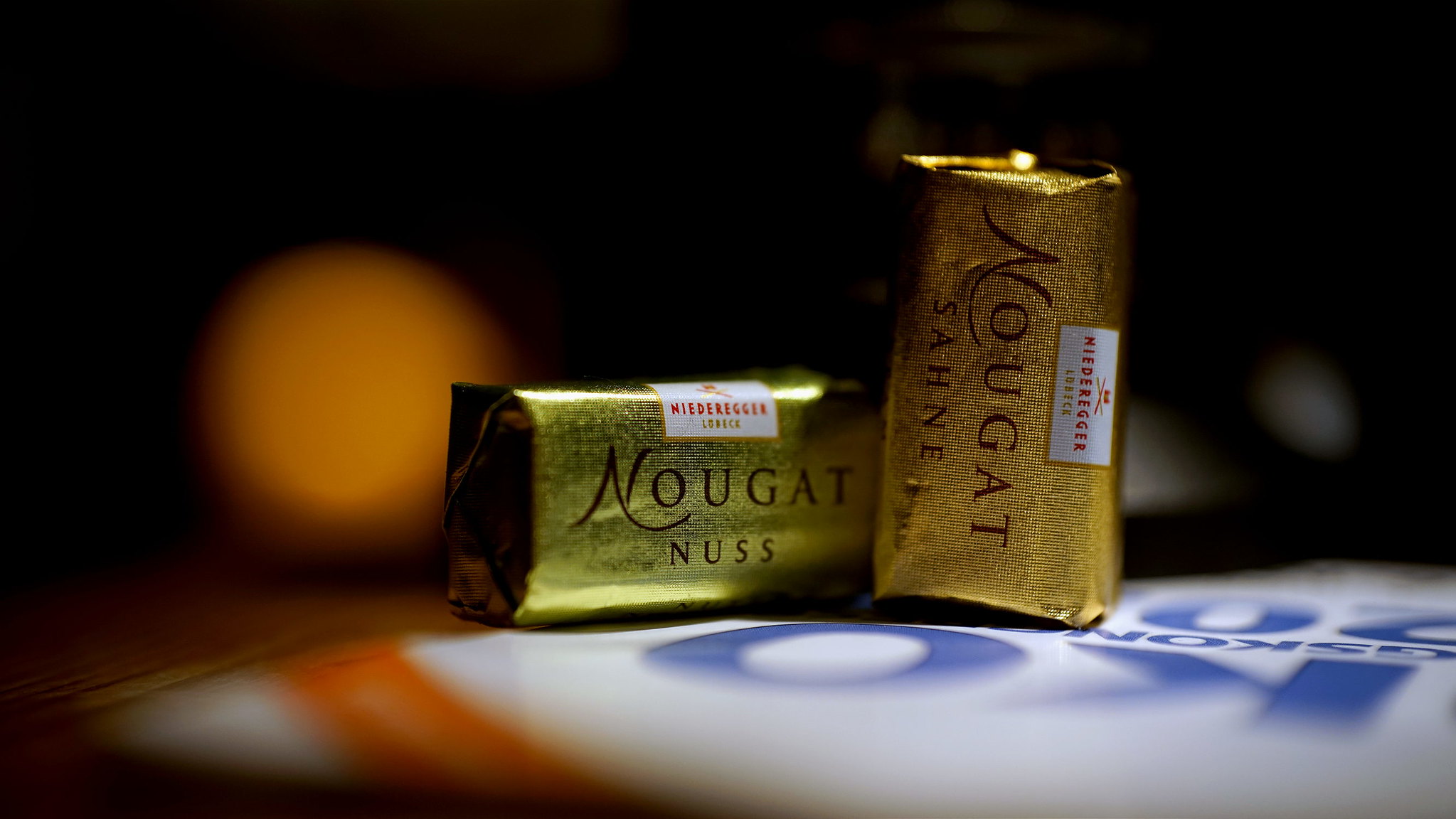The image is a horizontally aligned rectangular picture featuring two clearly visible pieces of candy, possibly nougat or chocolate, wrapped in gold foil. One piece of candy is placed horizontally, while the other is standing vertically. Both candies have brown lettering on the wrappers; the horizontal one reads "NOUGAT NUSS" with "NOUGAT" in larger letters and "NUSS" in smaller letters underneath. The vertical one reads "NOUGAT SAHNE." Each wrapper also has a small white label with red print saying "Niederegger," accompanied by an indistinguishable gold word underneath. The background of the image is blurry, predominantly solid black on the upper part, indicating a low-light or nighttime setting. On the left side, there's a vague gold object. The candies rest on a blurry surface that seems to be a table or desktop, possibly with a sign underneath it featuring white with large blue letters.